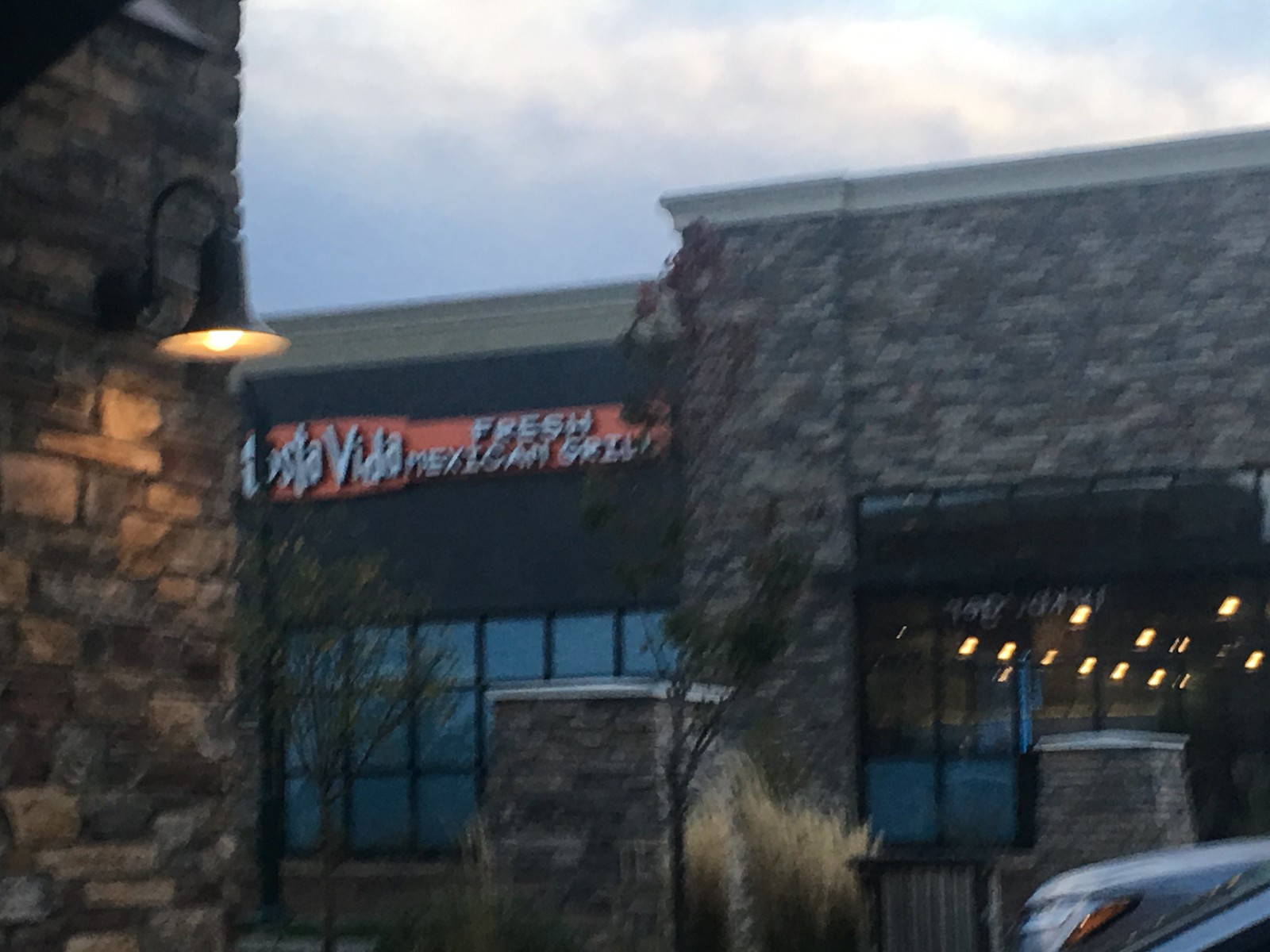The image depicts the front of a restaurant building made of bricks in various shades of gray, tan, and possibly darker brown. Prominently displayed on the left side of the building is a sign with an orange background and white lettering that reads "Costa Vida Mexican Grill," though the first few letters are partially obscured. The sign is mounted on a black section of the wall. Below the sign, there are several square windows with window panes, through which the interior lighting of the restaurant is visible. Additionally, there is a light fixture outside the restaurant. To the bottom right of the photo, a small portion of a gray car, including its orange and white lights, can be seen. The image is somewhat blurry, and a black pole near the left side partially obstructs the view of the sign.